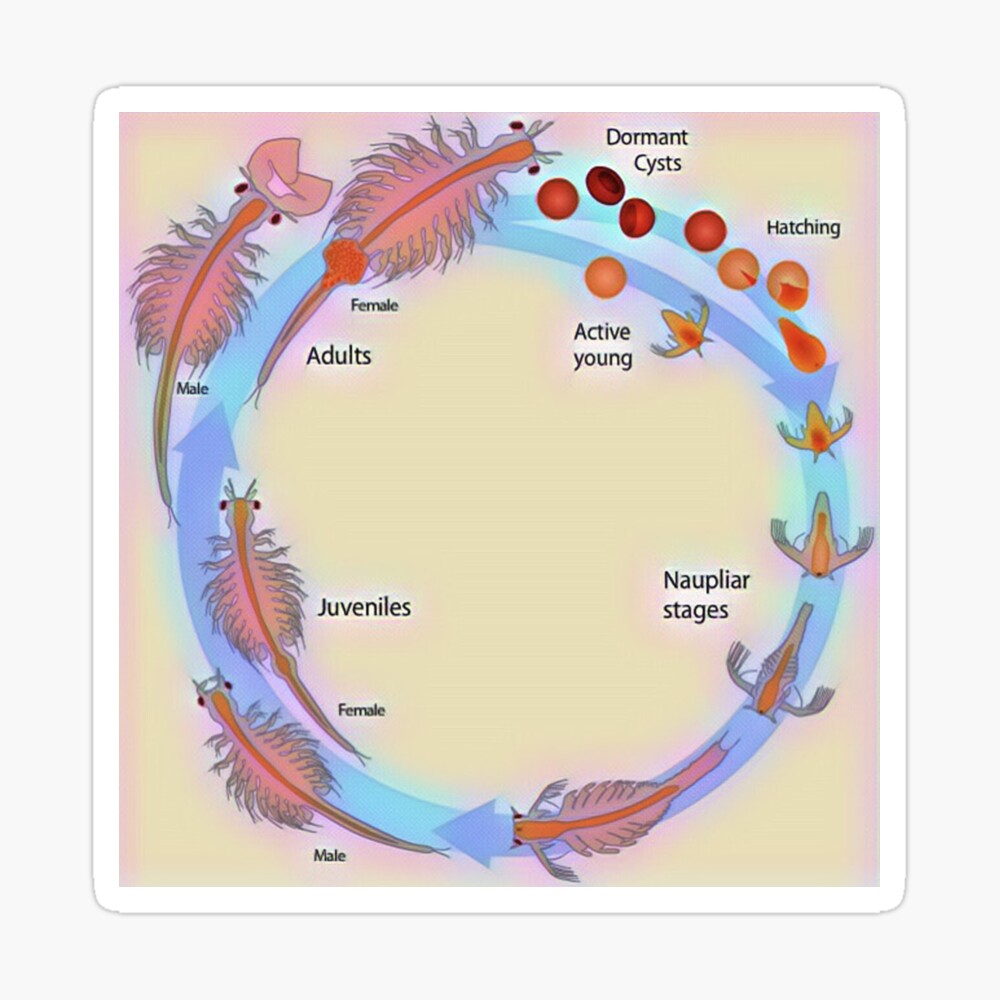The image is a vertically rectangular infographic designed for educational purposes, featuring a detailed lifecycle of an organism, possibly a mite. The central illustration is surrounded by a white border on a background that shifts between brown, yellow, and pink shades, giving it a cloudy appearance. Within the infographic, the lifecycle progression is depicted through blue arrows with a gradient from cyan to purple, showing various developmental stages from Dormant Cysts, resembling acorns, to Active Young, Hatchlings, Nauplier Stages, Juveniles, and finally to Adult Males and Females. The mature adults are illustrated with multiple legs, a simple digestive tract, protruding eyes, and long tails. The primary colors used in the artwork include gray, black, orange, and shades of red, enhancing the visual distinction of each life stage.